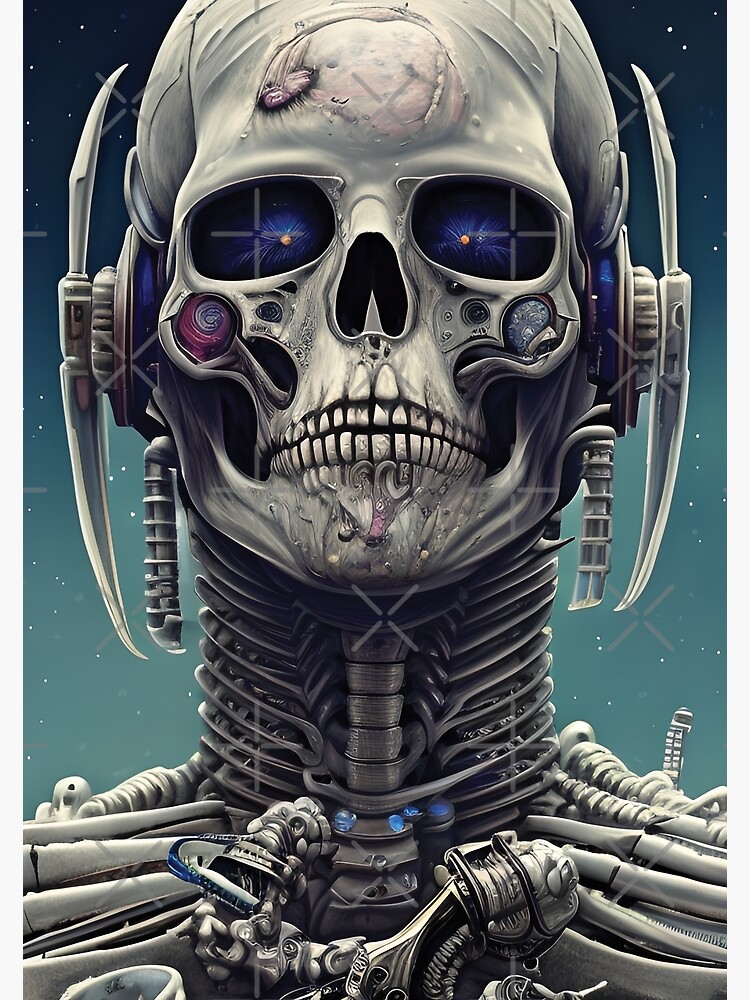This digital pixel art illustration features a predominantly teal gradient background, transitioning from light teal at the bottom to dark teal at the top, adorned with delicate white star-like specks. Dominating the frame is an intricate, metallic android-like figure designed to resemble a futuristic skeleton. The figure boasts a shimmering silver to light blue hue, reflecting a metallic sheen throughout its form.

The head of the android is skull-like, complete with hollow eye sockets, nose cavities, and rows of exposed teeth. Inside the eye sockets, there appear to be swirling galaxy designs, punctuated with faint yellow dots. The cheekbones also display intricate spiraling galaxy patterns. A distinctive feature is a pink round mass located on the top of the skull, accompanied by a purple, tumor-like protrusion. Extending from the sides of the head, headphone-like devices with larger discs attached give the appearance of advanced auditory equipment.

The android's neck reveals a complex structure, resembling an assembly of narrow metal rings layered horizontally, with a prominent trachea-like metal tube running along the front. Horizontal metallic structures mimic clavicles, enhancing the mechanical anatomy. The shoulders and upper torso are crafted from shiny, interlocking metal pieces, forming a sophisticated exoskeleton that highlights the fusion of robotic and skeletal elements in this striking artwork.